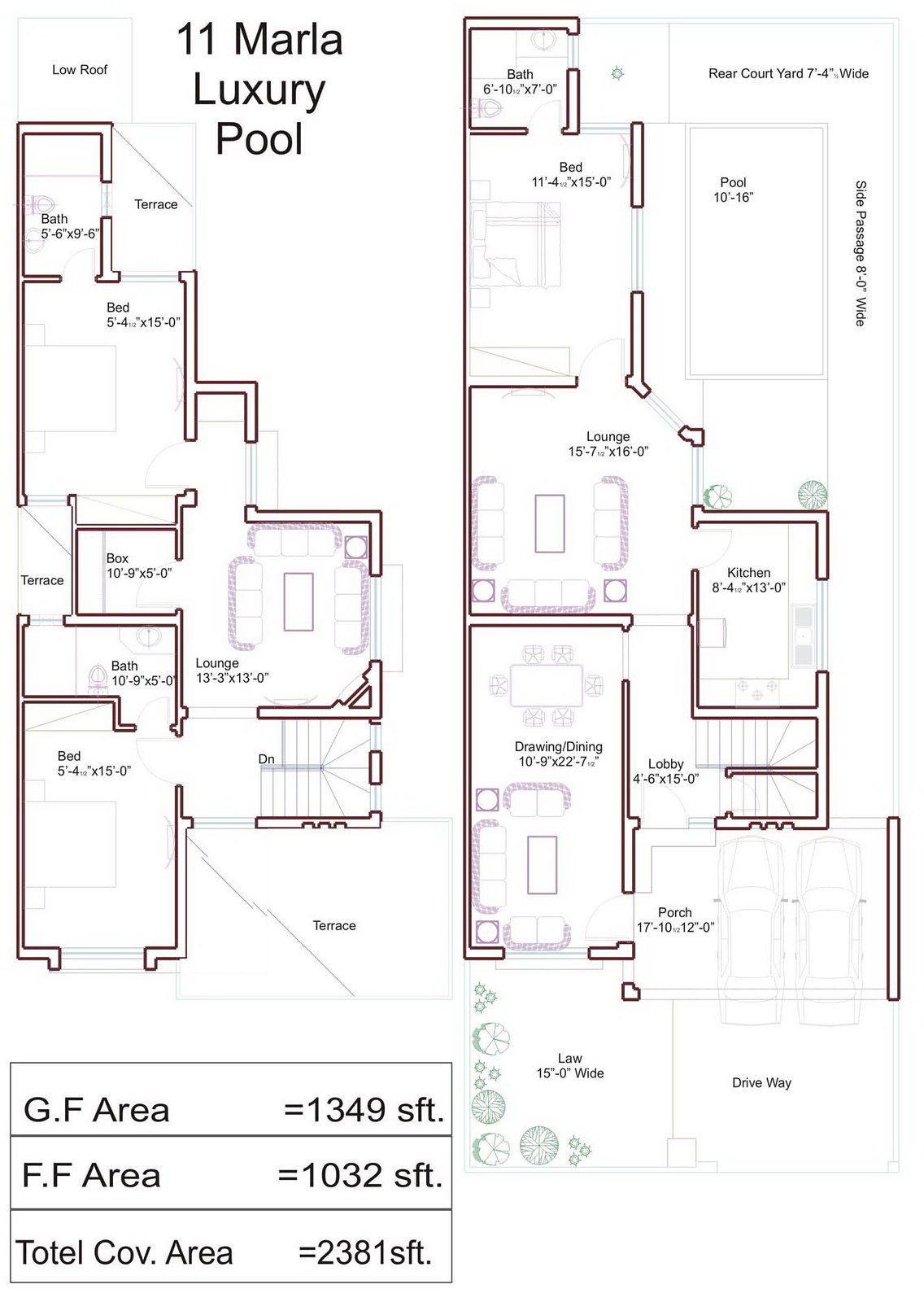This detailed floor plan depicts a luxurious, multi-level apartment. The layout is divided into two sets, possibly indicating different floors, and includes a driveway, where cars are visibly parked. 

Upon entering the apartment, one is greeted by a lobby area that provides access to a set of stairs leading upwards. Adjacent to the entryway is a spacious living room, followed by a dining room. Continuing through the apartment, there is a porch that offers additional outdoor space. 

The first floor features a well-equipped kitchen and a lounge area furnished with three couches—two placed opposite each other, and one positioned at the back—accompanied by two tables, two side stands, and a coffee table. Walking further leads to a pool area, which has a side passage for convenient access. Adjacent to this pool area is a rear courtyard and a bedroom furnished with a queen-size bed, a dresser, and an attached half-bathroom, equipped with a counter and a toilet.

The upper floor includes a large bedroom with an en-suite bathroom, another lounge area, and several terraces that offer additional outdoor living spaces. This floor also features a second bedroom with an attached bathroom and a terrace. 

The overall area of the apartment is highlighted with a luxurious 11 Marla Pool. The ground floor measures 1,349 square feet, while the upper floor covers 1,032 square feet, bringing the total covered area to 2,381 square feet.